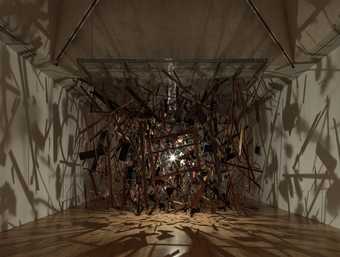The image captures a dimly lit, indoor space resembling a gallery with a creepy, otherworldly ambiance. Its eerie atmosphere is accentuated by the tall ceilings, painted in dark hues that contrast with the cream-colored walls. The wooden floor adds a sense of warmth that is juxtaposed by the sinister setting. The centerpiece of the scene is an intricate 3D sculptural installation that emits an unsettling glow from a central light source, casting chaotic shadows of floating black shapes and geometric patterns across the room. These shadows create an illusion of random shapes and lines, giving an impression of things suspended mid-air. The overall effect is reminiscent of a scene from a horror movie or an avant-garde art display, filling the space with an aura of mystery and unease.